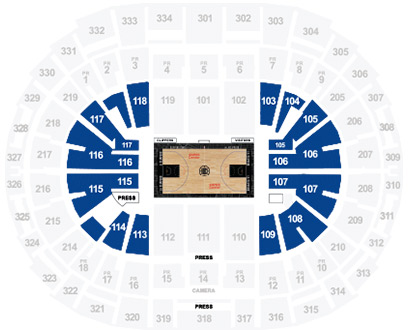The image depicts a detailed seating chart of a basketball stadium against a white background. At the center of the image, a small illustration of the basketball court reveals the wooden floor. Surrounding the court, rectangular sections represent various seating areas. Notably, the sections situated adjacent to the hoops on both the right and left sides are highlighted in blue. Each section is labeled with numbers for easy identification, such as 103, 104, 105, 106, 107, and 108. Directly beneath the basketball court, section 111 is prominently featured, followed by sections designated for the press, labeled PR 14, and an area marked for cameras and additional press coverage. The seating arrangement extends outward in three concentric levels of rectangles, encapsulating the entire stadium layout.